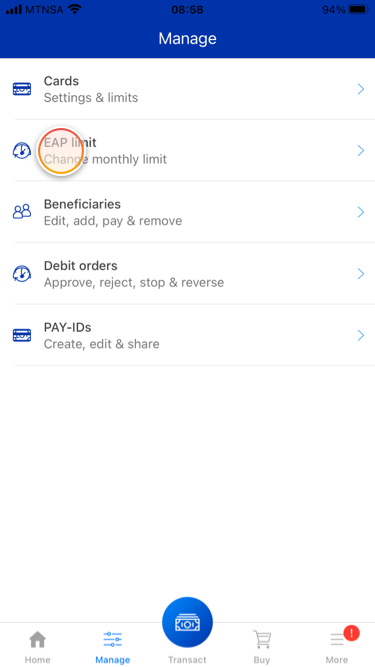Top left of the screen shows full cellular bars indicating strong signal strength, followed by the label "MTNSA." Next to it, full Wi-Fi bars are displayed. In the top center, the time reads 8:58, and the top right corner shows a battery indicator at 94% capacity. Beneath the time, the word "Manage" is visible.

As we move down the screen, there's a section titled "Card Settings," which includes options for viewing and configuring limits. An image of a card is shown on the right side, with arrows pointing right next to various sub-options such as "EAP Limits," "Change Monthly Limits," "Beneficiaries," and "Edit, Add, Pay, Remove." Next to the "Beneficiaries" option, there is a small icon representing two people.

Further down, there's another section for "Debit Order Management" with choices to "Approve," "Reject," "Stop," and "Reserve" debit orders, marked with the same icon as the EAP and pay sections. The "Pay-IDs" section offers options to "Create," "Edit," and "Share," which shares the same icon as the card image.

At the bottom of the screen, there's a navigation bar with options labeled "Home," "Manage," "Transactions," and "Buy & More." The "More" option has a notification indicator.